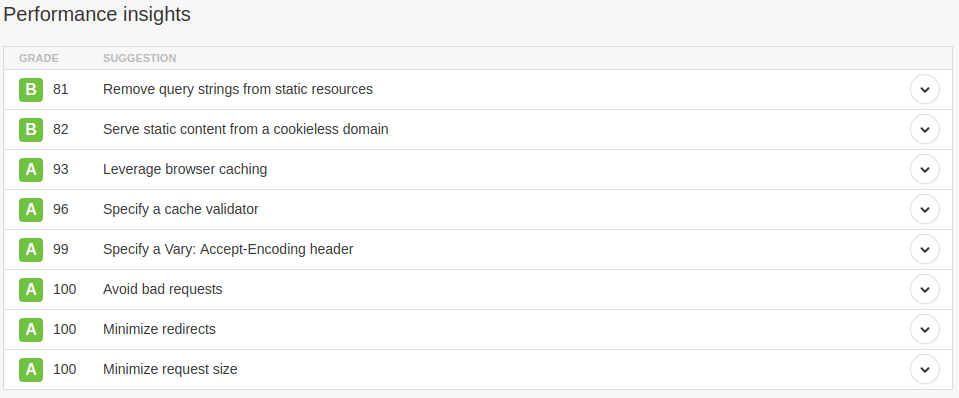The image showcases a performance evaluation screen titled "Performance Insights" presented in a simple, clean format. The top section of the screen features a black header with "Performance Insights" displayed prominently in a large font. Below the header, the screen is organized into columns. The first column heading is "Grade," followed by "Suggestion," with each entry clearly separated by lines.

The performance grades listed include both an alphabetical grade (A or B) and a numerical score adjacent to it, presumably representing the performance score. The suggestions for improvement are listed next to each grade. Here are the details:

- **B, 81**: Remove query strings from static resources.
- **B, 82**: Serve static content from a cookieless domain.
- **A, 93**: Leverage browser caching.
- **A, 96**: Specify a cache validator.
- **A, 99**: Specify a Vary: Accept-Encoding header.
- **A, 100**: Avoid bad requests.
- **A, 100**: Minimize redirects.
- **A, 100**: Minimize request size.

On the right side of each suggestion, there are interactive arrows that can be clicked, though their function is not specified in the description.